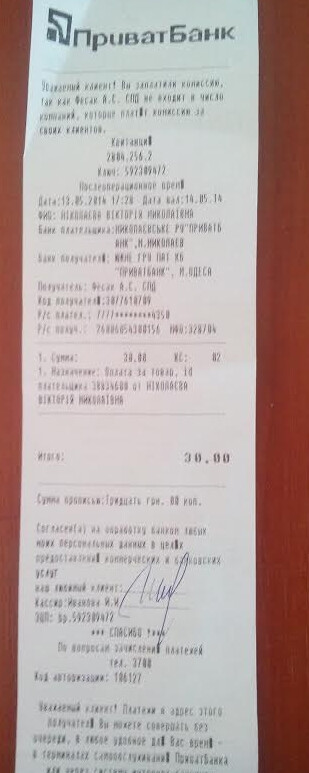The image showcases a white receipt placed on a reddish-brown, hard, flat surface that appears to have a wood grain pattern, though the pattern is only visible at the left and right edges due to the crop of the picture. The receipt is written in a language that is not easily identifiable and is quite blurry, rendering the letters difficult to read. At the top of the receipt, there are some numbers and detailed information, although they are not clearly legible. One of the few readable elements is a total amount listed as 30.00. Towards the bottom of the receipt, there is a section with additional information and what appears to be an actual signature, though again, the specific details are not discernible due to the blurriness of the image.